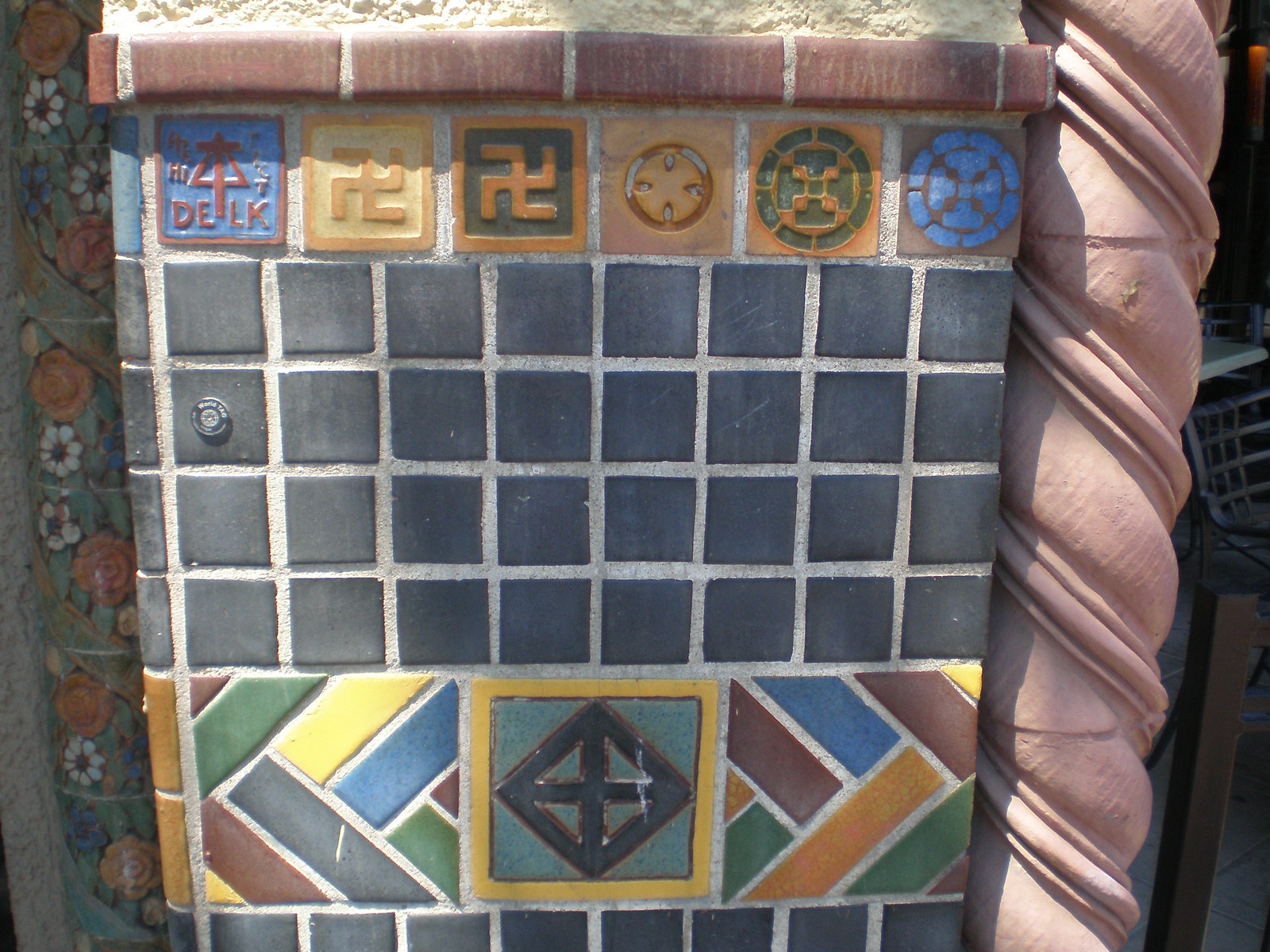This photo captures a detailed and colorful wall, possibly part of a historic or old building. The left edge of the wall features a vertical pattern of orange, white, and green flowers. Central to the image is a rectangular or almost square tiled section with diverse designs. At the top of this section, brick-colored tiles are arranged horizontally. Below these bricks are six square tiles, each about 5 inches by 5 inches, featuring various symbols and colors. The first tile has a blue background and is framed in red, with a cross over a triangle and the word "Delk" underneath. Following this, two tiles exhibit swastika symbols – one on a yellow background with a darker yellow frame, and another on an orange and green background. 

Next, there is a tile with a circle that has four lines around it in orange and terracotta tones. The subsequent tile, also in orange and green, contains a circle with a cross inside. The final tile in this row is framed in brown and blue. Below this row of tiles are smaller black squares, and at the very bottom is a vibrant tile featuring various geometric shapes in a mix of yellow, blue, black, green, burgundy, white, and orange colors. On the right side of the wall, a twisted, pink-colored vertical line resembling a swirl or a twisted clay rope adds to the intricate design of the wall.